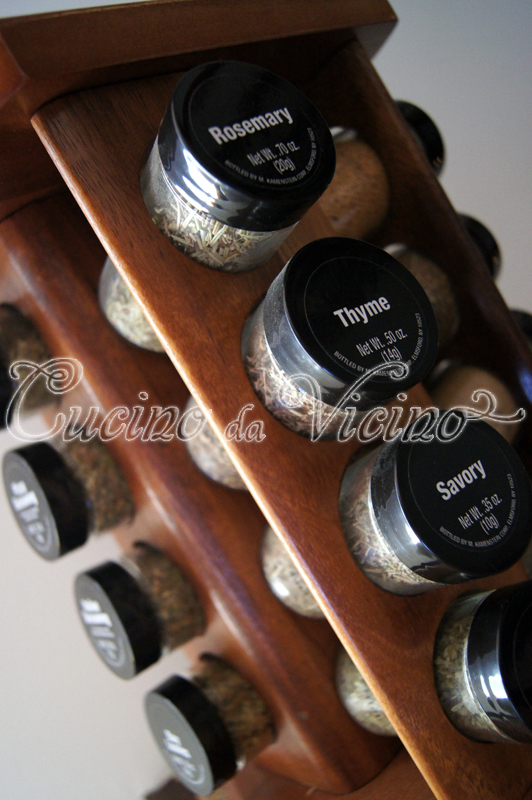This is a detailed picture of a wooden spice rack stained in a dark brown color, sitting on a kitchen counter against a white wall. The spice rack is in the shape of a cylinder, designed to be rotated, revealing multiple sides with cut-out circles to hold spice jars. The angle of the photo shows the spice rack tilted at a 45-degree angle, giving a diagonal view. Each jar is made of clear plastic with black lids that feature white writing indicating the spices. The visible labels are rosemary, thyme, and savory, each revealing the green contents inside. The rosemary has a net weight of 0.30 oz, the thyme 0.50 oz, and the savory 0.35 oz. Though there are other jars on the blurred out opposite side, those specific spices are not identifiable in the picture.